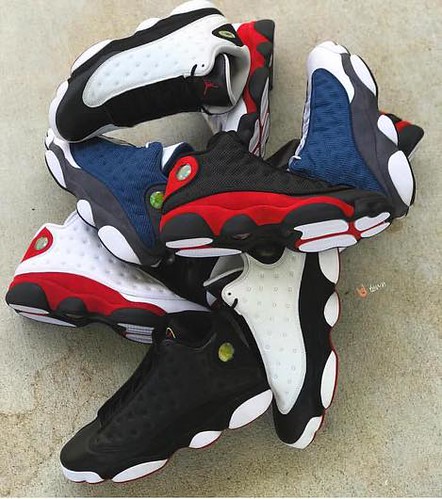The image depicts a chaotic arrangement of eight running shoes scattered across a light greyish-brown concrete floor. Starting at the bottom left, there is a black running shoe with white soles, followed by a white shoe with black lines and protruding white rubber soles. Centered in the middle is a black and red running shoe with white bottom soles and a hint of black edging. To its right lies a blue shoe with a black and white sole, with an identical pair nearby. At the top, a white running shoe features a black lining, while to its far left another white shoe is adorned with small indented holes and highlighted by red and black lining above white soles. Each shoe has a black and white base where colors such as red and navy blue are also visible, suggesting they are part of a coordinated collection, possibly for an advertising campaign. The diverse colors include navy blue, regular blue, black, and white, and the shoes appear to share a consistent tread pattern, though the brand remains unidentified.